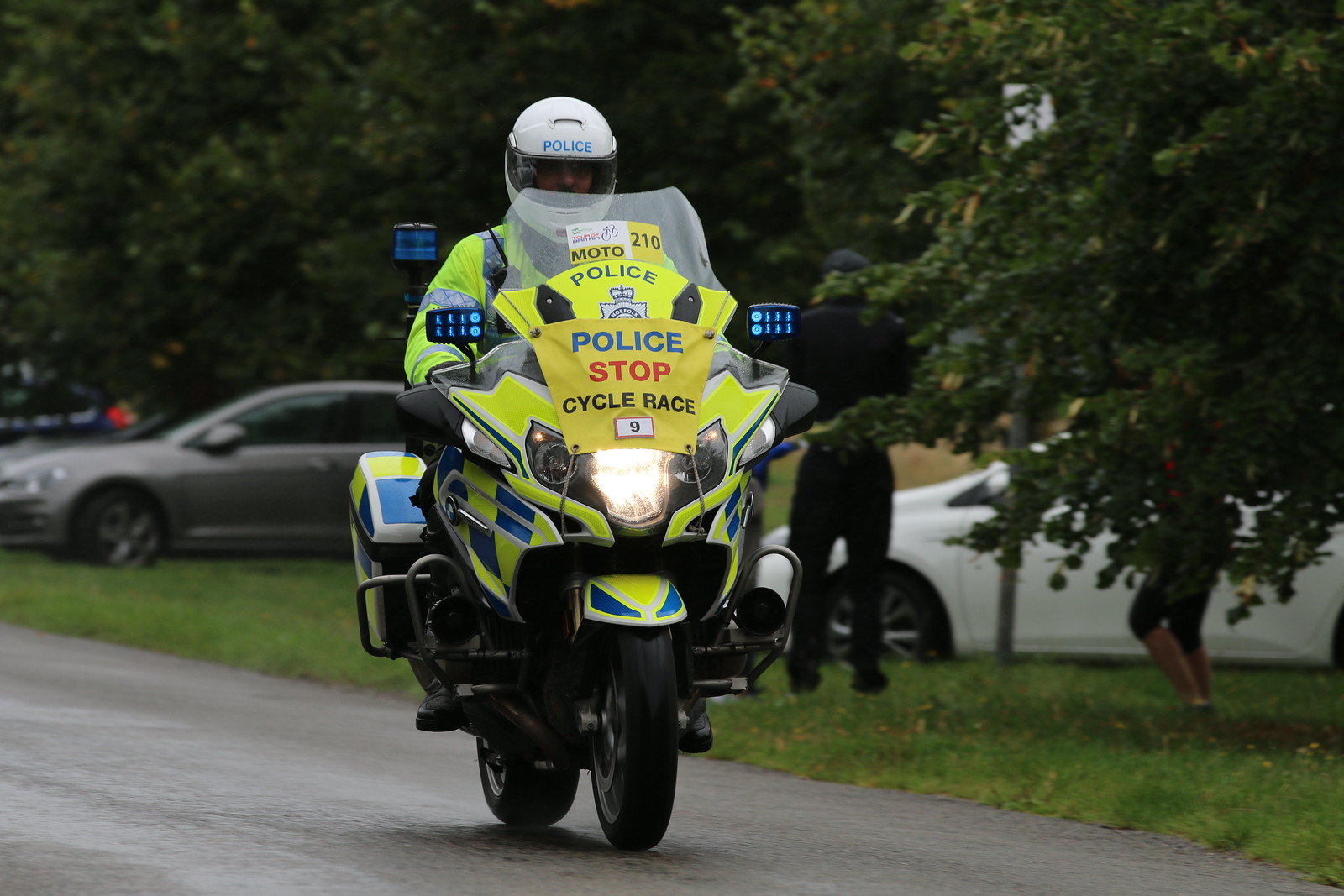This image captures a UK police officer riding a green, yellow, and blue police motorcycle slowly down a wet concrete street. The officer, dressed in a yellow jacket and a white helmet marked with "POLICE" in blue text, navigates the bike with his hands firmly on the handles. Positioned prominently on the motorcycle's windshield are the labels "Police," "210MOTO," and "Police Stop Cycle Race," emphasized by blue and red text. Surrounding the scene, several cars, including a white one and a gray one, are parked on an adjacent grassy area. A couple of people, clad in black outfits, stand near these cars, with one man partially obscured by a tree, observing the vehicles. The backdrop is filled with lush trees, suggesting a midday setting under cloudy skies. The lights on the police motorcycle are vividly blue, and the back of the bike features a square storage container.